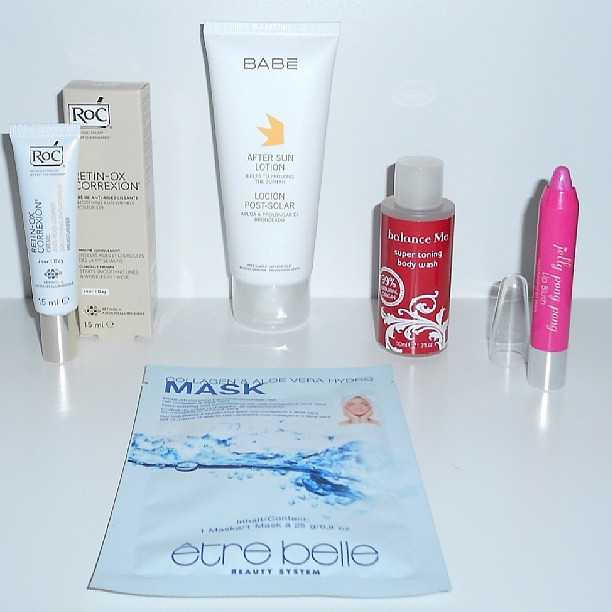This photograph captures a close-up view of a collection of beauty products arranged neatly on a glossy white counter, likely in a bathroom. The background is a pure white wall. In the foreground lies a blue flat package labeled "Collagen Aloe Vera Hydro Mask" featuring a splash of water design and the brand name "Etra Belle Beauty System." Directly behind this mask, prominently centered, stands a large white tube reading "Babe After Sun Lotion" with orange detailing. To its left, there is a white bottle with a silver cap labeled "Rock Retinol OX Correction," accompanied by its gray box packaging. On the right side, a plastic bottle with a red label reads "Balance Me Super Toning Body Wash." Additionally, a pink crayon-like item, possibly a lipstick or lip pencil, also appears on the right side, capped with a plastic cover. The overall arrangement showcases a variety of products including lotions, body washes, and skincare items, all skillfully spaced against the pristine white counter and wall.